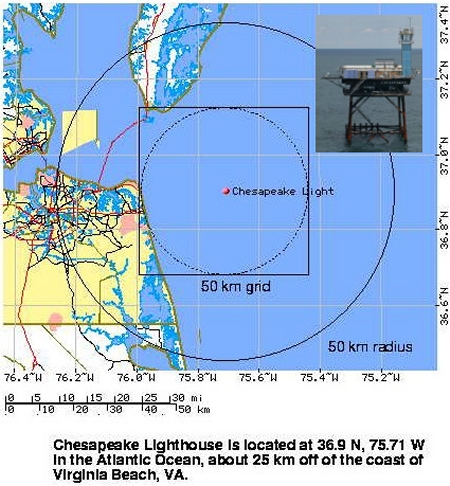This image illustrates a GPS map centered on the Chesapeake Lighthouse, marked by a red dot labeled "Chesapeake Light." Dominating the middle of the map, Chesapeake Lighthouse is accurately positioned at 36.9 N, 75.71 W in the Atlantic Ocean, approximately 25 kilometers off the coast of Virginia Beach, Virginia. Concentric circles emanate from the lighthouse, denoting a 50 km grid and a subsequent 50 km radius, which are clearly marked. The left side of the map features minimal land detail, primarily showing a peninsula extending from the land mass. Degrees of longitude and latitude are precisely delineated on the bottom and right-hand side of the image, ranging from 76.4 W to 37.4 N. In the top right corner resides a photograph, presumably of the lighthouse, though it bears a resemblance to an oil rig, with the text "Chesapeake Light" beside it.